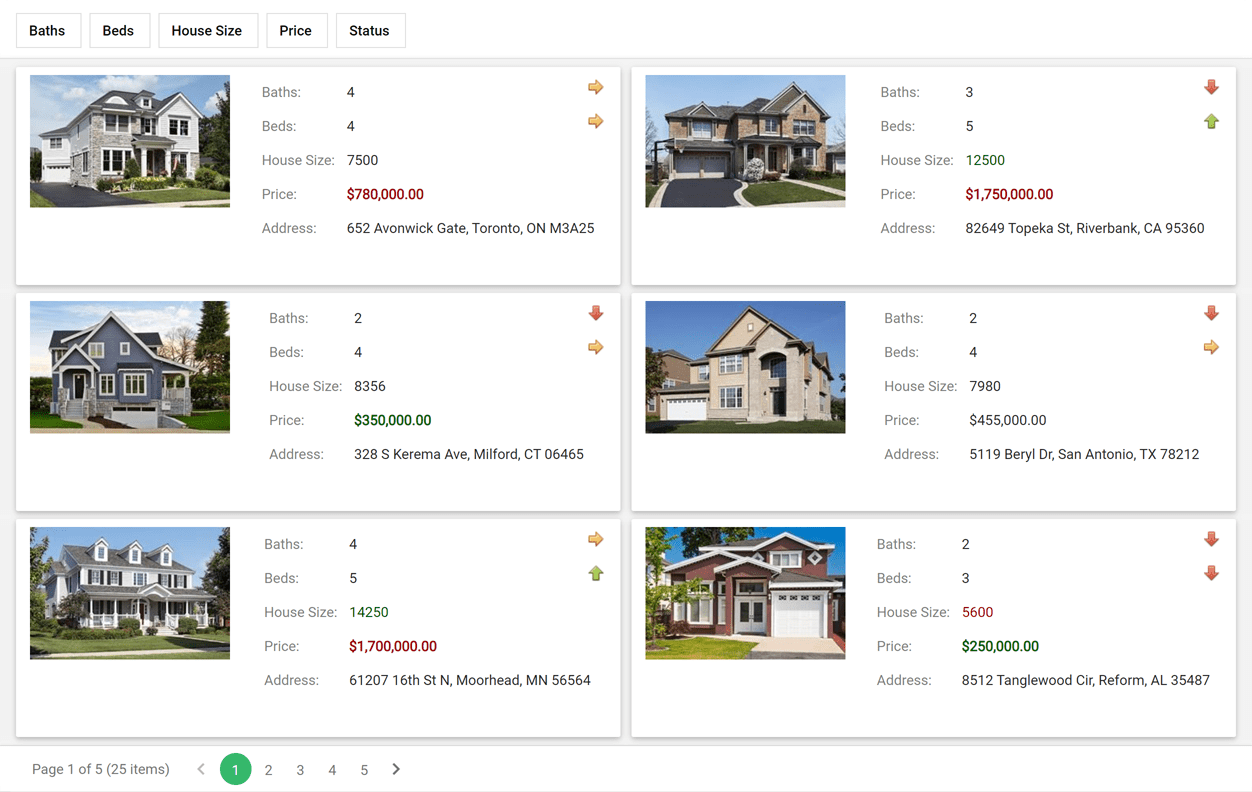The image showcases a series of real estate listings featuring various houses and their details. 

1. The first house is priced at $780,000, offering 4 bedrooms and 4 bathrooms, with a total house size of 7,500 sq ft.
2. The second house is listed at $350,000, featuring 4 bedrooms and 2 bathrooms, with a house size of 8,356 sq ft.
3. The third house has a price tag of $1,700,000, including 5 bedrooms and 4 bathrooms, and boasts a house size of 14,250 sq ft.
4. The fourth house is priced at $1,750,000, offering 5 bedrooms and 3 bathrooms.
5. The fifth house is listed for $455,000, featuring 4 bedrooms and 2 bathrooms.
6. The sixth house is priced at $250,000, featuring 3 bedrooms and 2 bathrooms, with a total house size of 5,600 sq ft.